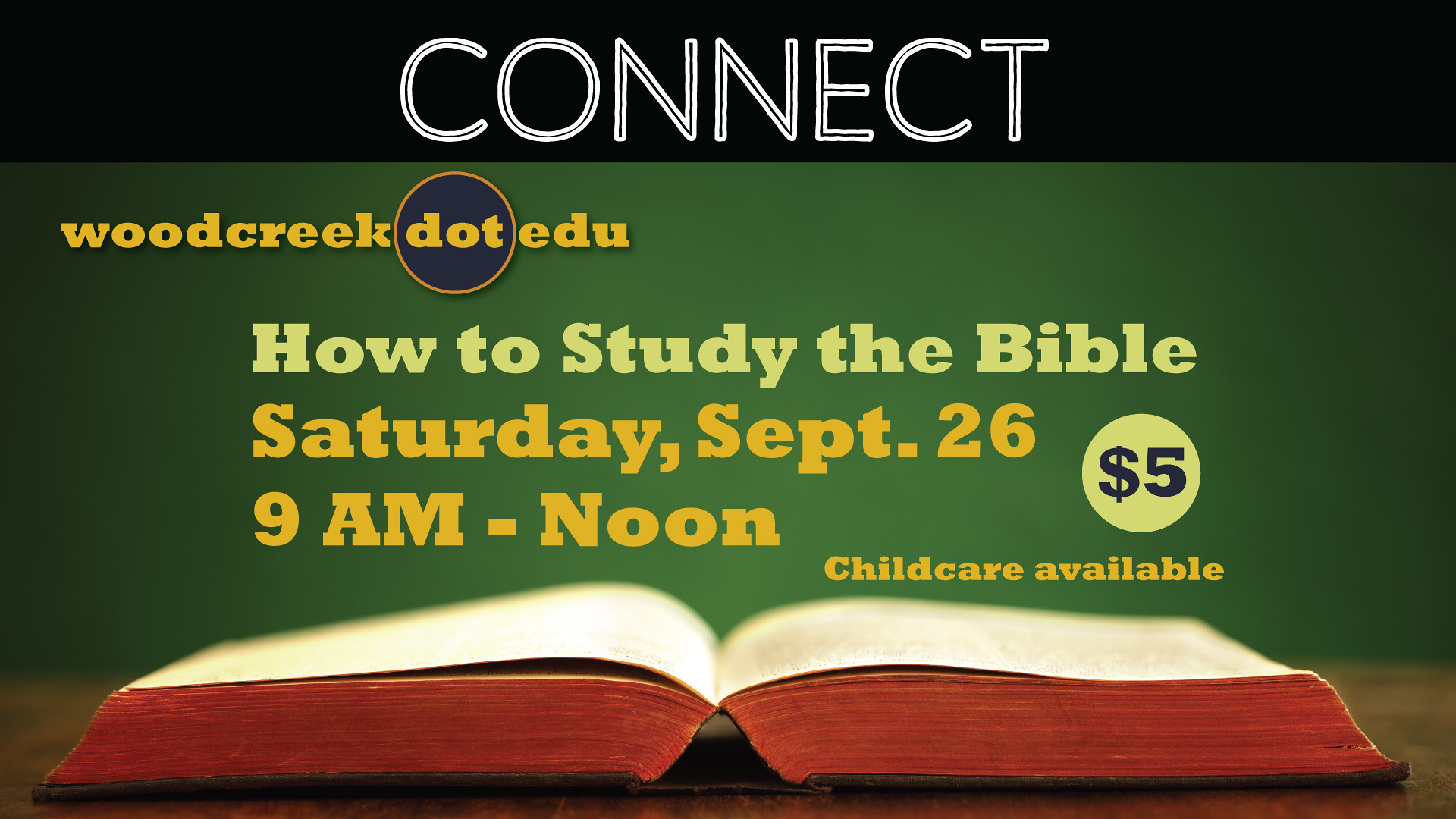This image is an advertisement for a Bible study event hosted by a church. The background of the advertisement is predominantly green, with a black bar at the top featuring the word "Connect" in white letters. Below this, the text "woodcreek.edu" is prominently displayed. The event details read: "How to Study the Bible, Saturday, September 26, 9 a.m. to noon." An orange-colored circle with a $5 fee is clearly visible, and the advertisement mentions that childcare will be available. At the bottom of the image, there is an open Bible with red-edged pages laying flat on a wooden table. The various text elements are formatted in shades of light green and yellow, providing a visually cohesive look against the dark green backdrop.